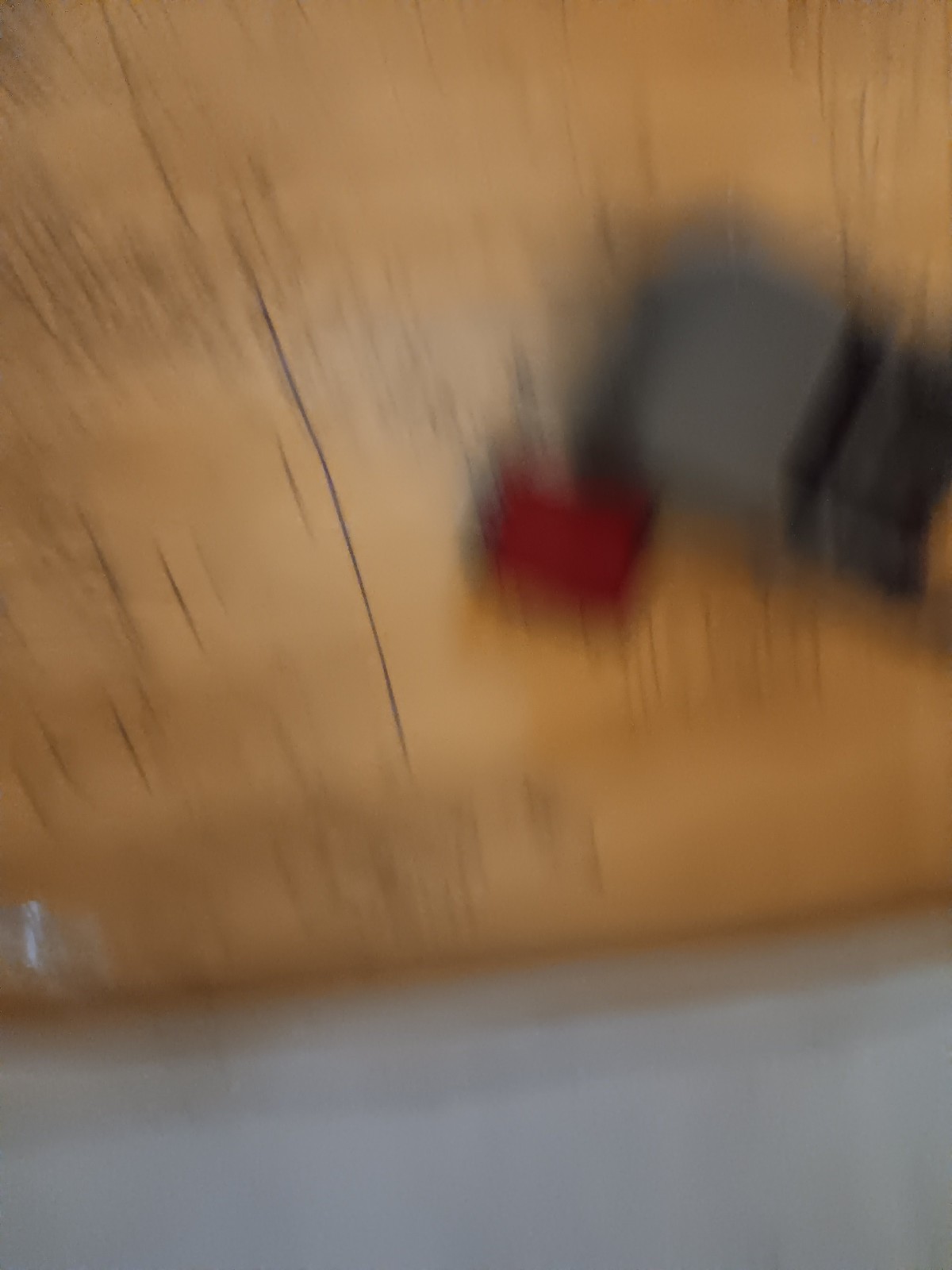The image is extremely blurry and lacks clear orientation, leaving it uncertain if it is upside down. The lower third of the image has a light gray, almost white background, which seamlessly transitions into a dark, muddy brown line. The remaining two-thirds are dominated by a yellowy pine color, possibly representing a floor or ceiling, adorned with indistinct black lines. Towards the top-right corner, there is a square consisting of two different shades of gray, beside which sits a small red block. The overall composition suggests the objects might be positioned on a piece of cardboard, viewed from above. However, due to the heavy blurriness, the actual subjects remain indiscernible.